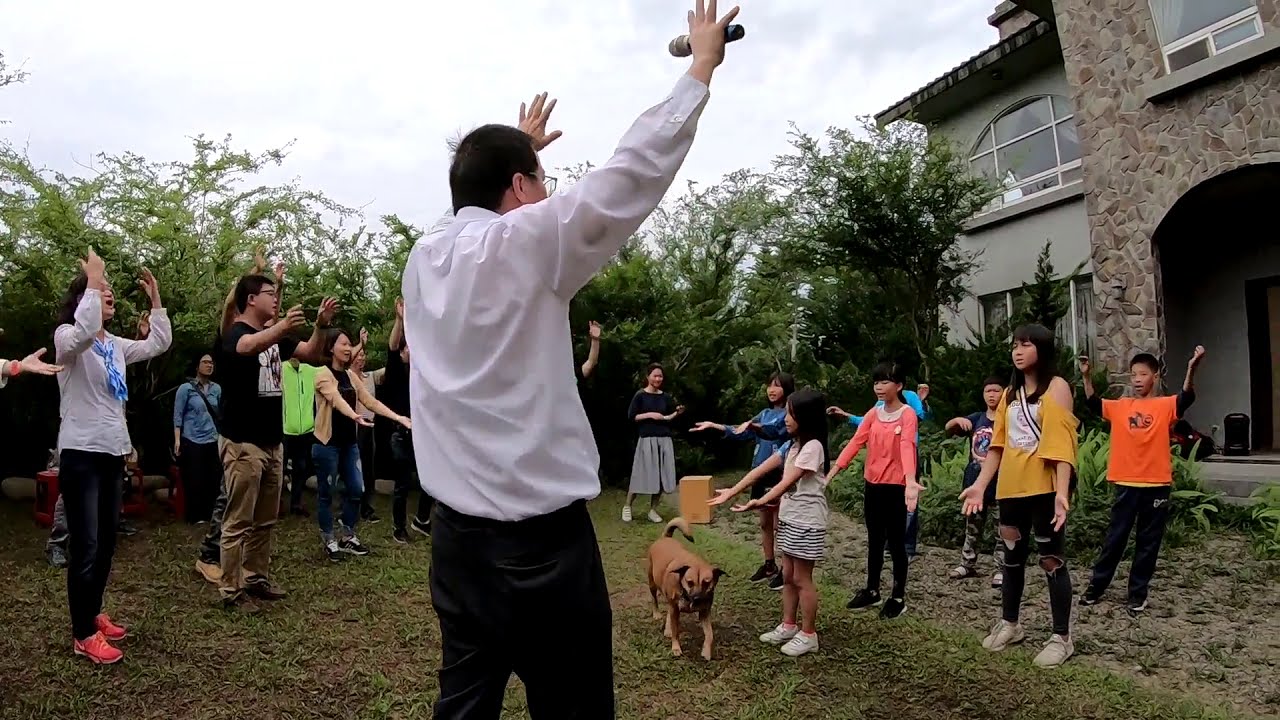In this horizontally aligned rectangular photograph, a group of people is gathered on a green, albeit muddy, lawn in the backyard of a large stone house, partially visible with its front of gray brick and large windows. The group is split into two distinct clusters, with adults on the left and children on the right, all facing each other. A large brown dog with a long tail walks towards the viewer in the middle of the scene. Central in the foreground stands a man wearing a long-sleeved white button-down shirt and black slacks. With short brown hair and glasses, he holds a microphone in his right hand and has both arms raised above his head, seemingly giving commands. The children to his right, dressed in bright shirts of yellow, orange, white, and blue, mimic his gestures, possibly playing a game like "Simon Says." The adults behind the children also have their hands raised, mirroring the man’s pose. The sky above is mostly cloudy with a mix of bright white and gray clouds, and trees form a natural backdrop, framing this lively gathering.